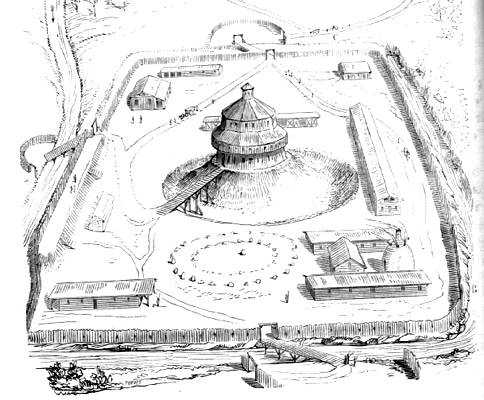This pen and ink drawing offers a detailed overhead view of an enclosed, historical fortress or village. Central to the composition is a prominent cylindrical structure, reminiscent of a tower or pavilion, featuring a ramp leading up to it and a cupola at its peak. Surrounding this central structure are various buildings, including rectangular stables or barns, arranged within a wooden stockade. 

The enclosure is composed of wooden or straw-like materials, and the layout displays clear pathways lined with rocks, creating circular patterns around the central structure. The entire area is encased by a substantial fence, with gates and bridges providing access across what appears to be a moat—likely indicating an additional layer of defense. Beyond the stockade, there are also trees and a body of water, possibly a lake or river, which enhances the medieval or rustic aesthetic of the scene. The drawing, executed on white paper, aesthetically straddles the line between a conceptual illustration and a historical sketch, capturing the essence of a fortified, ancient settlement.